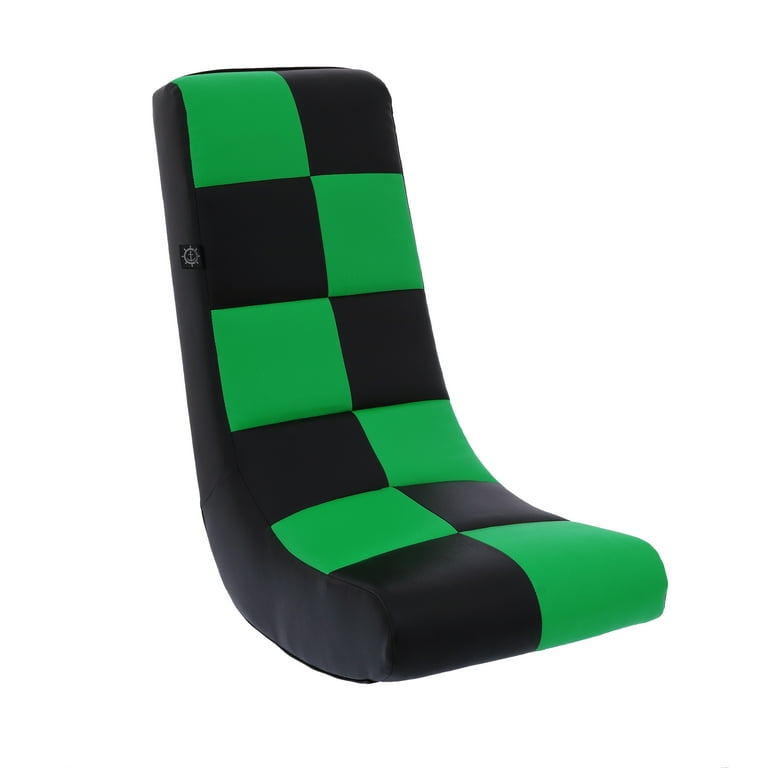This is a color photo of a gaming chair designed for seating directly on the ground. The chair has a unique and vibrant design featuring alternating rows of black and green checkered squares: green-black, black-green, repeated in sequence. It is L-shaped and the sides are solid black. The chair appears soft and cushioned, suitable for comfortable seating during gaming sessions. Notably, there is a black and white tag at the top side of the chair with an image resembling a ship's wheel with an anchor in the center; it contains no text. The chair includes integrated speakers on its sides to enhance the gaming experience. The photo is taken against a plain white background, making the chair's details stand out vividly.